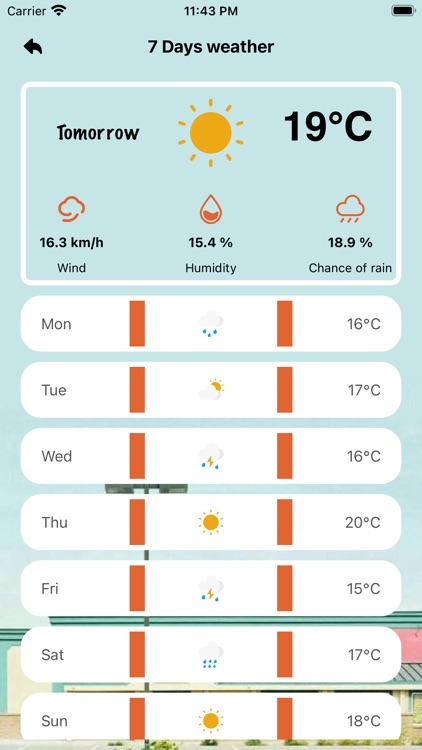The image is a detailed screenshot of a weather app. The background features a light blue color, likely representing the sky at the specified location. At the very top, the menu bar displays "carrier," suggesting it's a sample display, along with full Wi-Fi signal strength, the time (11:43 PM), and a battery at 100%.

Centrally positioned below the time, the app text reads "Seven Days Weather," accompanied by a back arrow with a curved tail. A prominent panel outlined in a rounded white rectangle provides specific details for "Tomorrow." This includes an icon of a yellow sun and a temperature of 19 degrees Celsius. Additionally, it notes that the wind speed will be 6.3 kilometers per hour, humidity at 15.4%, and a chance of rain at 18.9%, each iconically represented by a cloud with a tail for wind, a water droplet for humidity, and a cloud with rain lines for rain.

The weather forecast for the upcoming days is also shown:
- **Monday:** 16 degrees Celsius with rain, indicated by a rain cloud icon.
- **Tuesday:** Partly cloudy with a temperature of 17 degrees Celsius.
- **Wednesday:** Thunderstorms expected with a temperature of 16 degrees Celsius.
- **Thursday:** Sunny with a temperature of 20 degrees Celsius.
- **Friday:** More thunderstorms are forecasted, with a temperature of 15 degrees Celsius.
- **Saturday:** Rain anticipated with a temperature of 17 degrees Celsius.
- **Sunday:** Sunny with a temperature of 18 degrees Celsius.